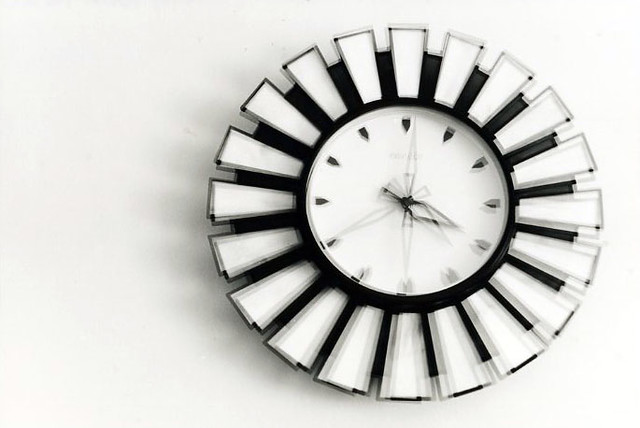This image depicts a unique and artistic clock hanging on a smooth, off-white colored wall. The clock, predominantly white, is circular with a complex design that extends beyond its center. The clock face itself is plain, missing traditional numbers and instead featuring black diamond-like shapes where the numbers would usually be. The clock hands, which are oblong and diamond-shaped, appear in multiple positions, creating an illusion that makes telling the exact time difficult. Surrounding the clock face are multiple rectangular extensions resembling sun rays or petals of a flower, outlined in black. These elements create an alternating pattern with the black background visible between them, adding to the clock’s intricate and somewhat confusing appearance.